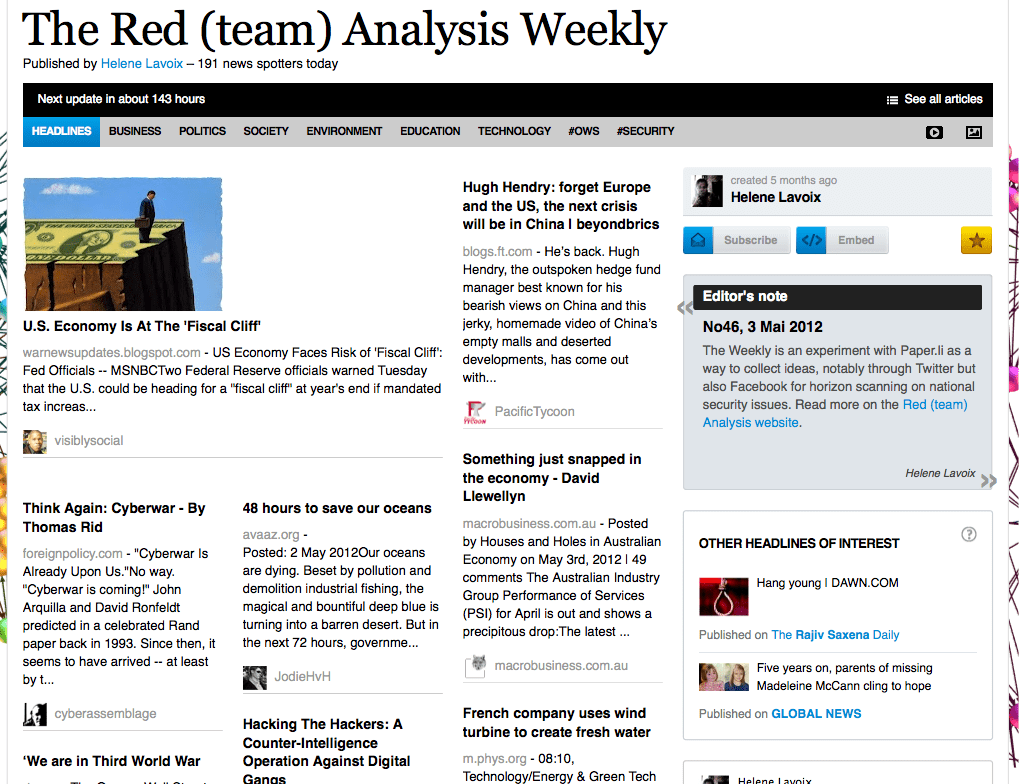At the top of the image, black text reads "The Red Team Analysis Weekly, published by Helene LaVoie - 191 News Spoiler Today." Below this, a black box displays a message stating "Next update in about 143 hours" and an option that says "See all articles." Beneath the black box, there is a toolbar with various categories: Headlines, Business, Politics, Society, Environment, Education, Technology, CWS, and Security.

Directly below the toolbar is an image showing a man dressed in a business suit, holding a briefcase as he stands precariously on the edge of a cliff. The cliff is uniquely topped with the face of a dollar bill, symbolizing financial peril. The caption superimposed on the image reads: "U.S. economy faces risk of official cliff. Federal Reserve officials warn that the U.S. could be heading for an 'official cliff' at year's end due to mandated tax increases." The sources cited include "Fed officials," "MSNBCT," and the "Federal Reserve."